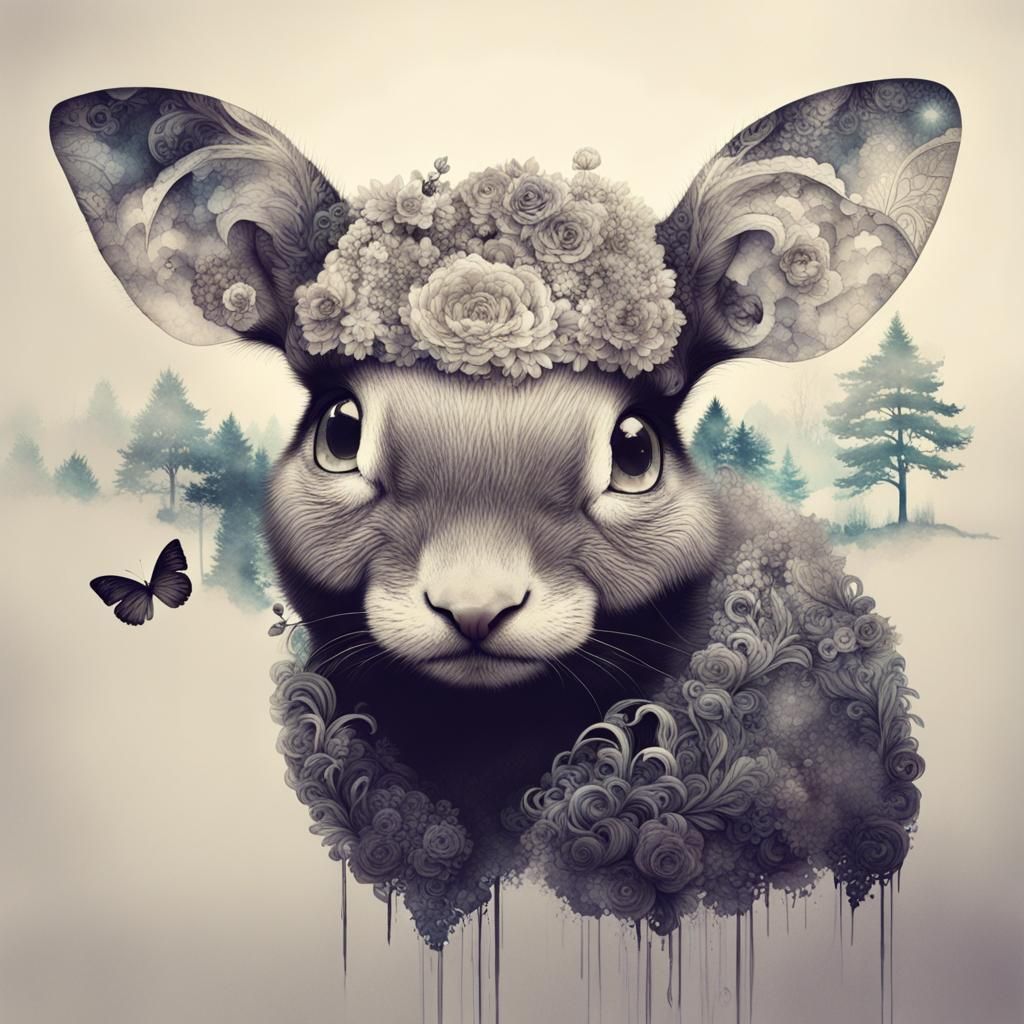The artwork depicts a highly stylized rabbit-like creature, primarily illustrated in grayscale with intricate floral patterns. The rabbit's head and shoulders are prominently featured at the center of the canvas, with its detailed face gazing forward, exhibiting light-colored, reflective eyes. Its fur is rendered in various shades of gray, and the ears are adorned with elaborate floral and sky patterns. Crowning the rabbit's head is an ornate hat composed of gray flowers.

The creature's body appears to be formed from intertwining vines and gray flowers, which extend and drape downward. Surrounding the rabbit's figure are additional plant elements, contributing to the organic, nature-inspired theme. In the background, a series of tree-covered, fog-obscured pine trees add depth and texture to the scene, painted with subtle hints of green. The overall background transitions from a gradient tan color at the center to darker shades towards the edges, culminating in a near-black at the corners, creating a vignette effect.

To the left of the rabbit, a black and white butterfly adds a final touch of contrast and movement to the composition, enhancing the ethereal and dreamy atmosphere of the piece.